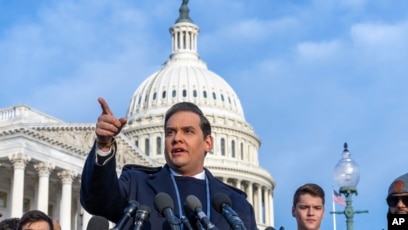This photograph captures a man, potentially George Santos, the former congressman under indictment, addressing the press in front of the Capitol Building's iconic white dome in Washington, D.C., with a deep blue sky and scattered white clouds as the backdrop. He is centrally positioned in the image, visible from the chest up, looking slightly to the left, and pointing with his right hand. He has short hair parted to the side, described variably as brown or black. He is dressed in a long-sleeve navy blue coat or suit jacket, layered over a white dress shirt and possibly a tie or vest. Surrounding him are five to eight microphones. Partially visible heads of other individuals, including a white man with brown hair and an African American man wearing sunglasses, are cut off at the bottom edges of the photo. A decorative green metal lamppost with a glass lamp, and what might be the Lincoln Memorial with its prominent white pillars, are present in the scene. The bottom right corner of the image features the "AP" logo, indicating it was taken by the Associated Press.